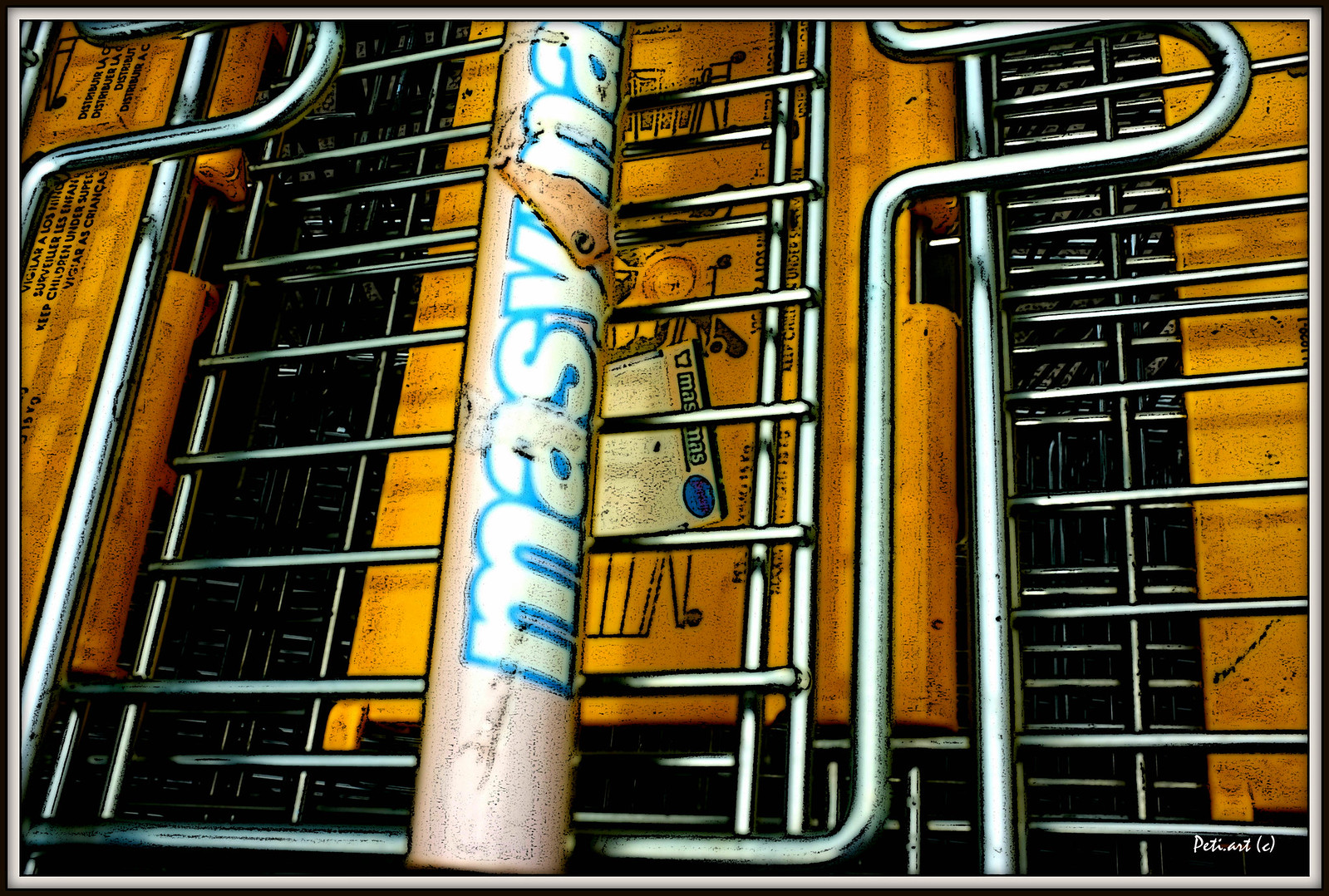The image is an extreme close-up of shopping carts nested together. At the forefront, there's a worn white painted metal pipe with blue text that seems to spell out "MASY MASY" though some of the letters are faded. This pipe is surrounded by a metal grate structure comprised of both horizontal and vertical shiny bars, likely stainless steel, with thicker bars running along the bottom and curving upwards. Behind the pipe, the shopping carts feature yellow rectangular panels, which act as dividers to prevent items from falling out. There's also signage on these panels displaying warnings about not letting kids stand in the carts. The backdrop includes additional sections of nested shopping carts, emphasizing the repeating pattern of the metal framework. The overall scene is set in what appears to be a grocery store named "Masi Mas."